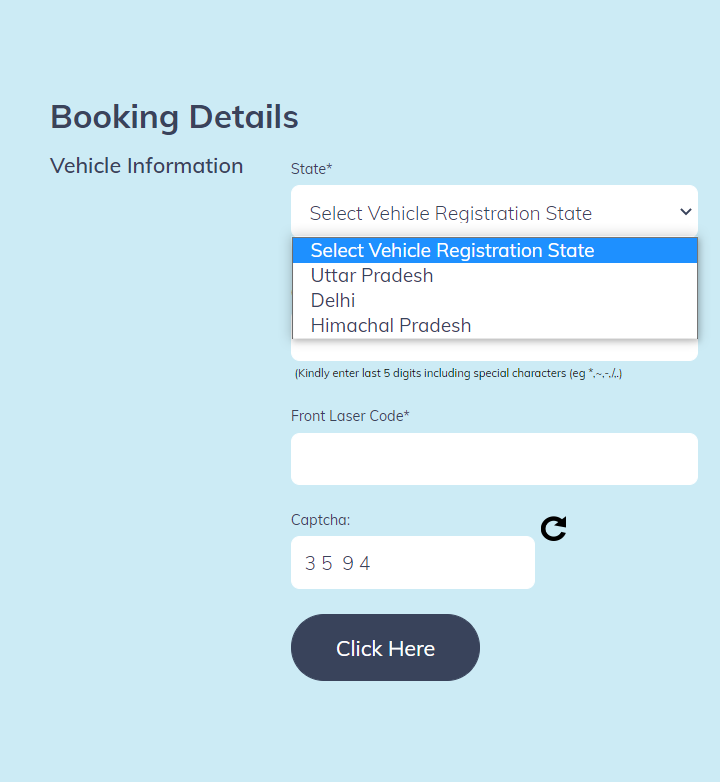This image displays vehicle booking details against a light blue background that appears almost white. The heading "Booking Details" is prominently shown in bold black font with both "B" and "D" capitalized. This heading is positioned approximately four spaces down and two spaces to the right from the left margin.

Directly beneath this heading, the text "Vehicle Information" is displayed in a smaller font. To the right of this text, there is a label saying "State" followed by an asterisk, indicating a required field. Below this, there is a white drop-down menu box labeled "Select vehicle registration state." Options available in the drop-down menu include "Andhra Pradesh," "Delhi," and "Himachal Pradesh."

Further down, additional input fields include a text box designated for the front license code, and a CAPTCHA box for verification purposes.